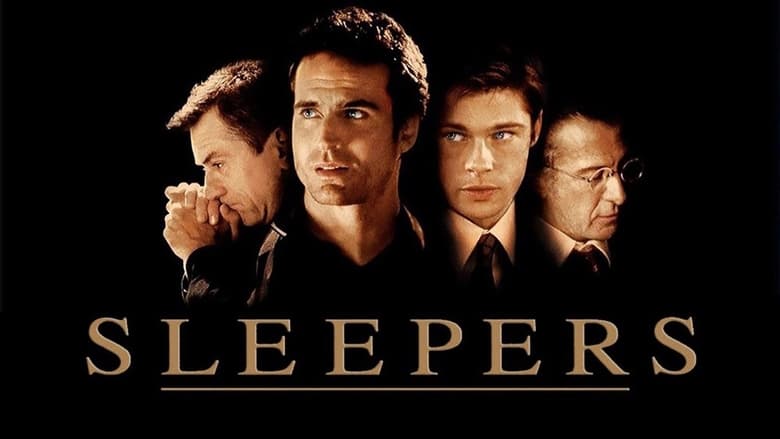The image is a movie poster for the film "Sleepers." The background is stark black, adding a dramatic flair, while at the bottom, the movie title "SLEEPERS" is prominently displayed in underlined gold, all capital letters. This poster showcases a lineup of four notable actors in the movie.

On the far left is Robert De Niro, characterized by his brown hair. His hands are clasped together and his face rests on them, conveying a very serious, perhaps concerning expression. Next to him is Jason Patrick, also with brown hair, who is slightly turned to the right, seemingly looking towards something beside him. 

To Jason Patrick's right stands Brad Pitt, youthful and gazing directly at the camera with a serious demeanor. Finally, at the far right is Richard Dawson, marked by his larger nose and glasses. He is looking downward with his head tilted, eyes closed, and an enigmatic smile on his face.

These actors are arranged to give a sense of cohesion and depth, each contributing a distinct expression and pose that hints at the complexity and gravity of the film's narrative.